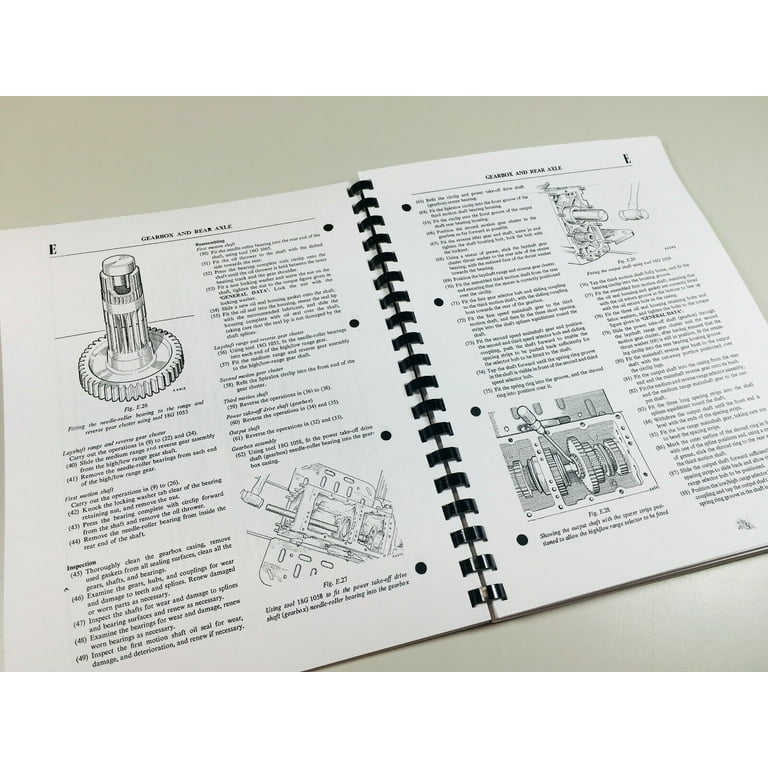This photograph captures an open manual lying on a white surface, specifically designed in a ring-bound booklet style. The binding features black plastic clasps running down the center, reminiscent of a notebook's metal spiral, but made of plastic. The two visible pages prominently feature the headings "Gearbox and Rear Axle" at the top. In the corners of each page, the letter "E" is printed. Both pages contain a detailed mixture of text and illustrations; the illustrations depict gear components, including a gear piece with a cylinder, among others. Each page is organized into two columns, with the text—although quite small—clearly providing step-by-step instructions on installation and usage, exemplified by phrases like "slide the medium range and reverse gear." The manual's overall design, featuring a combination of scientific graphics and detailed instructional content, suggests this might be an owner's or technical manual.